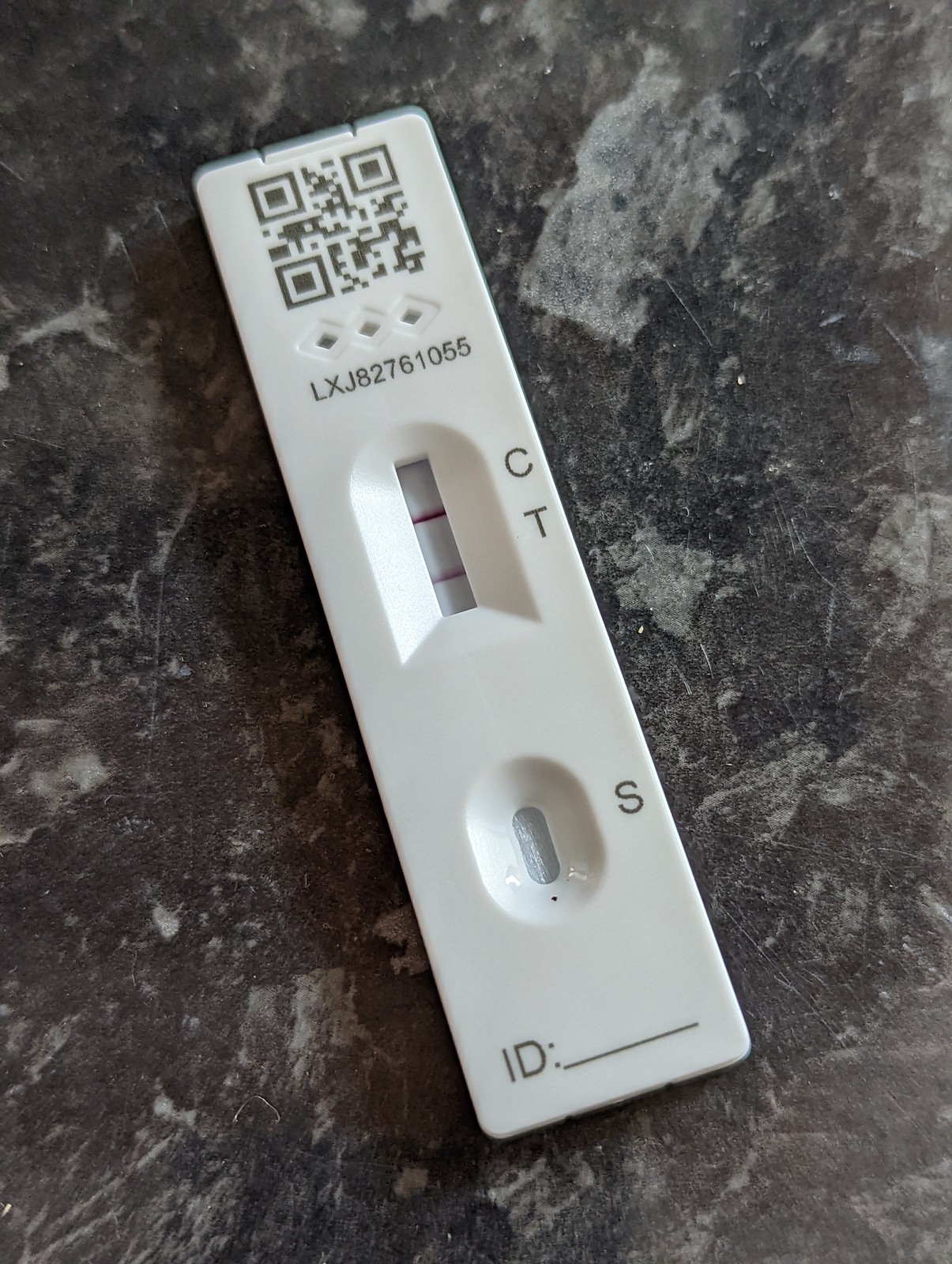In the image, there is a tabletop or background with a marbled appearance, predominantly featuring shades of black and light gray with some whitish tones, reminiscent of marble. On top of this marble-like surface, there's a white rectangular remote control. At the top of the remote, there's a black QR code in a square format. Below the QR code, three diamond-shaped engravings are present, with lights inside these shapes that appear to be turned off.

In the middle section of the remote, there's a long, vertically oriented, skinny rectangular screen displaying two purplish horizontal lights. These lights are separated by a small space. To the right of this rectangular screen, the letters "C" and "T" are printed in black, one above the other. Near the bottom part of the remote, there is a longer vertically oriented oval screen or light. To the right of this, the letter "S" is displayed in capital black letters. At the very bottom of the remote, the text "ID:" is printed in black, followed by a long underlined space, implying a place for an identification code or number.